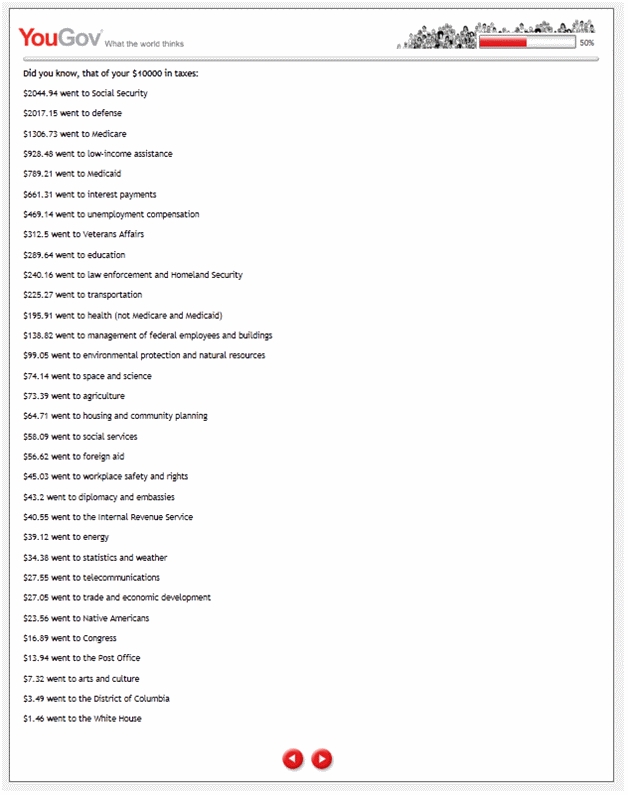In this image, there is a detailed breakdown of how tax contributions are allocated to various government services. The image appears to be from a webpage, possibly from YouGov, as suggested by the banner at the top which reads "YouGov" and includes their slogan "What the World Sees." The breakdown is presented in a clear and organized manner, illustrating how a hypothetical $10,000 in taxes would be distributed across different sectors.

- $2,044.94 is allocated to Social Security.
- $2,117.15 goes towards Defense.
- $1,306.73 is used for Medicare.
- $928.48 is directed to Low Income Assistance.
- $789.24, $929.48, and $501.70 are also noted for Social Security, indicating a possible repetition or emphasis on different allocations within the same sector.
- $929.21 is allocated to Medicaid.
- $661.31 goes to Interest Payments.
- $469.14 is used for Unemployment Compensation.
- $312.50 is directed to Veterans Affairs.
- $289.64 is allocated to Education.
- $240.16 goes towards Law Enforcement and Homeland Security.
- $225.27 is used for Transportation.
- $195.91 goes to Health, among other smaller categories.

The breakdown continues with other categories, providing a comprehensive view of how tax dollars are utilized by the government, ensuring transparency in public spending.